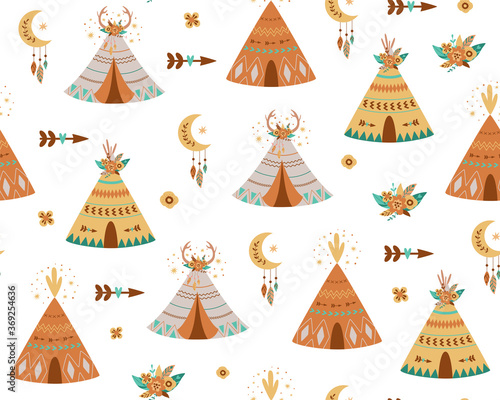This illustrated image, resembling a kid's wallpaper or a greeting card cover, features a white background with a pattern consisting of nine variously colored teepees scattered across it. The teepees, depicted in maroon, beige, white, and yellow hues, exhibit diverse details: some have brown and green stripes, others display turquoise and pink flaps or intricate designs like diamonds and antlers. There are maroon teepees with green dots and brown and yellow accents, white ones with antlers and diamond patterns, and yellow teepees adorned with intricate designs and green diamonds. Among the teepees, there are additional Indian artifacts including arrows, flowering plants, feathers, and crescent moons with colorful feathers hanging down. The moons feature gold writing with small stars inside and are decorated with brown and green feathers. The entire background of the image is white, emphasizing the vibrant illustration of the teepees and elements interspersed among them.